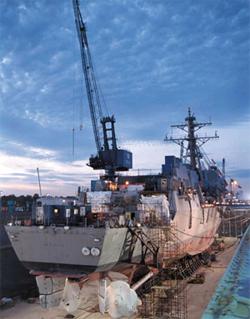This is an outdoor image of a large industrial ship, likely a cargo or military vessel, viewed from the back. The ship is situated on a concrete dock, not in the water, indicating it's in a shipyard or an industrial port setting. The ship features a tall mast with two extended arms and is primarily a concrete gray color with some black and green elements. Dominant colors in the scene are neutral, with the ship's gray hue prominently standing out. There is a significant silver crane positioned either on or behind the dock, possibly working on the ship. The background sky is filled with swirling, fluffy grayish-blue clouds, suggesting a stormy atmosphere or an early dawn setting, with streaks of purple and pink adding to the dramatic sky. No people are visible, but there are orange and yellow lights present. Additional colors in the scene include some brown tones on the dock and occasional green and blue hues. The sky predominantly features these muted colors, creating a tranquil yet industrial ambiance.